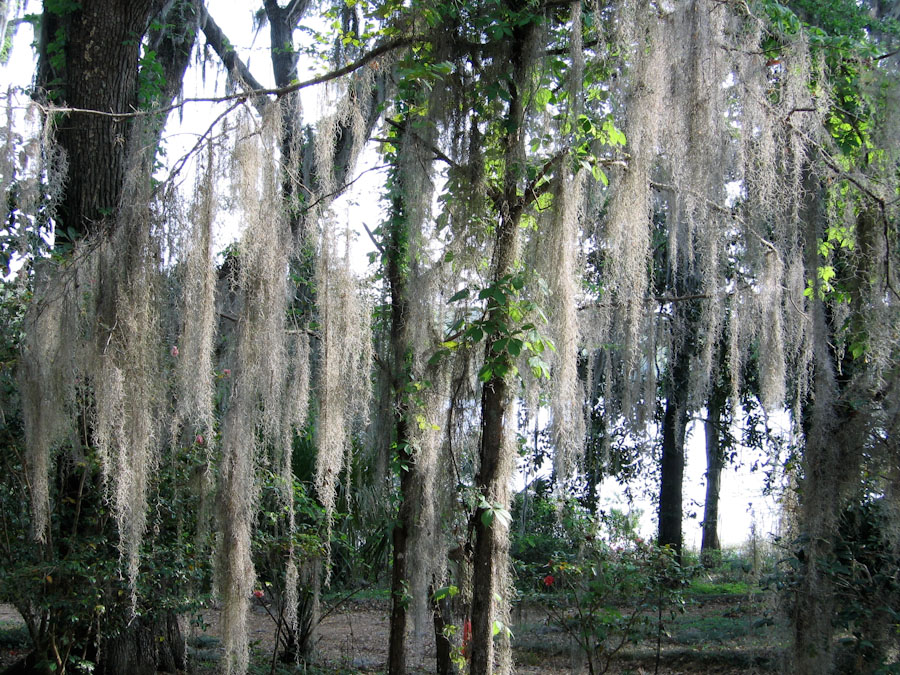The image showcases a tranquil early morning scene in a diverse forest setting. The landscape is dominated by numerous tree species, many with long, draping branches adorned with a peculiar, cottony white mesh material that hangs down, resembling filmy netting or soft fuzz. This white mesh is the most striking feature, standing out against the dull grayish color of the tree trunks and the various shades of green leaves, some of which appear vibrant where they catch the dappled sunlight filtering through.

The forest floor is primarily composed of brown dirt, sparsely covered with plant life, small shrubberies, and occasional flowers, hinting at a lively but undisturbed undergrowth. There is also a notable trail winding through, indicating that the area may see visitors from time to time, yet still retains a sense of serenity and peacefulness. On the right-hand side of the image, the forest appears to be adjacent to a calm lake, its surface incredibly smooth, reflecting the stillness of the morning. The sky above is a milky white, suggesting the early hours of the day before the sky fully brightens. The background shows a forested shore across the lake, completing the serene and picturesque scenery.